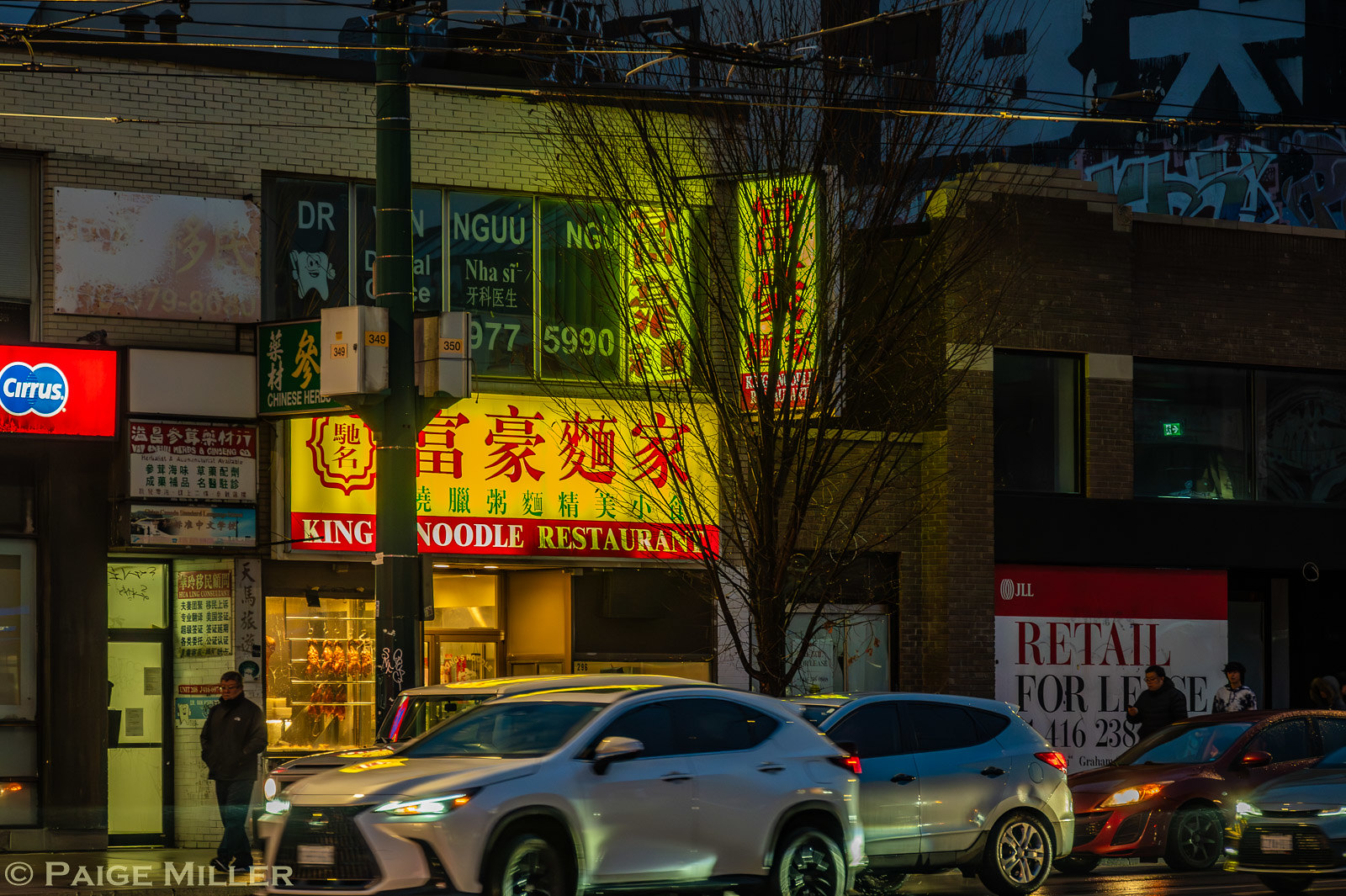This nighttime outdoor photograph captures a lively Chinatown street scene in a city. The foreground features cars parked along the street, with their headlights illuminating the road ahead to the left. The central focus of the image is a well-lit restaurant called King Noodle Restaurant, identifiable by its eye-catching yellow and red backward sign. Adjacent to it on the left, a smaller sign reads "Cirrus" in red and blue. A leafless tree with barren branches stands to the right of the restaurant, adding a touch of starkness to the scene. 

A man stands underneath the King Noodle Restaurant sign, while two other pedestrians walk past a storefront with a "Retail for Lease" sign in black text on a white background. Additionally, there is another person in motion on the street, creating a slight blur indicating movement. The photograph appears to be taken from across the street, providing a broad street view of the various businesses.

In the bottom left corner of the image, there is the text "Copyright Paige Miller," confirming the authorship of the photograph. This detailed street view encapsulates the nocturnal hustle and bustle typical of a Chinatown district.